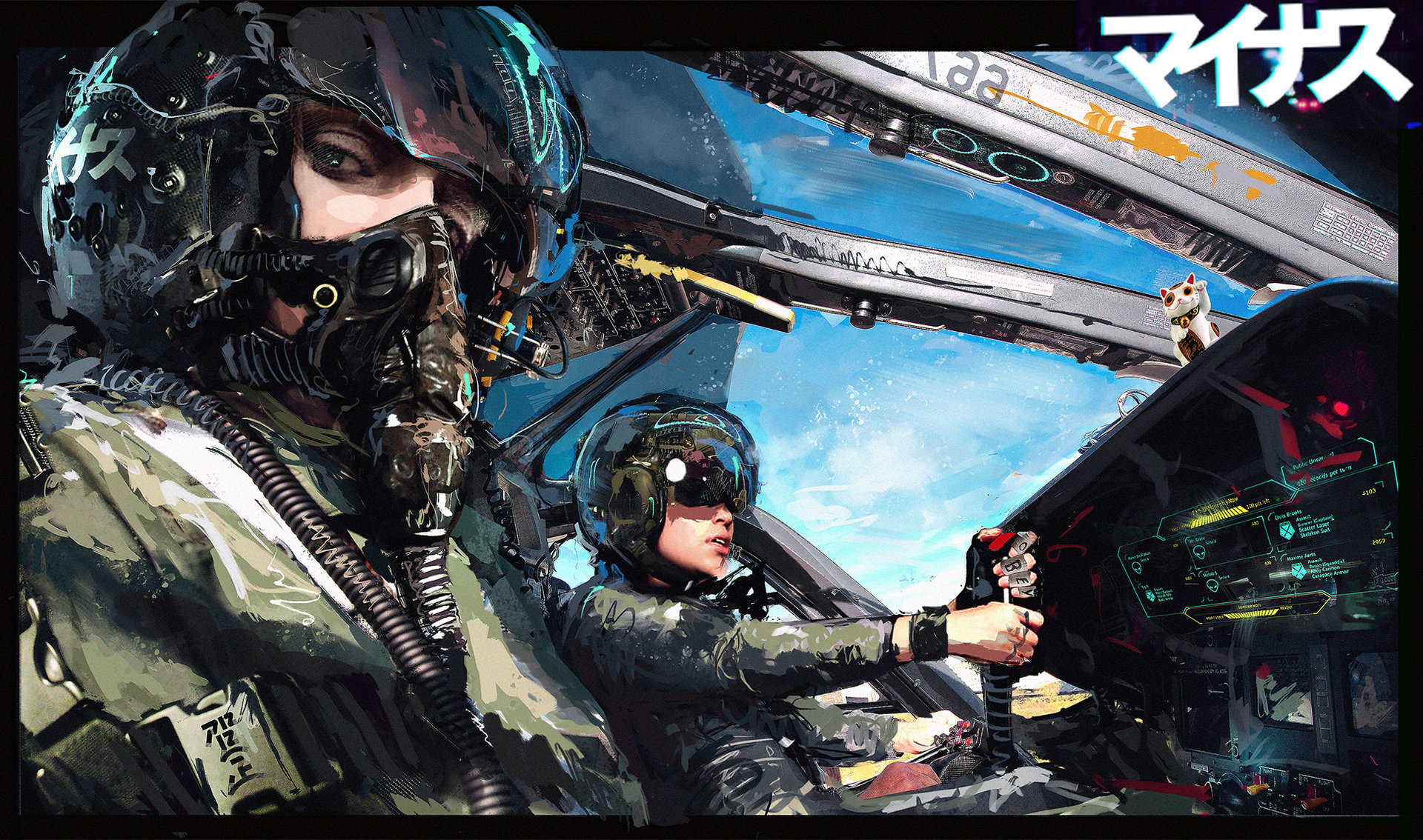The image depicts an intricate anime-style drawing of two individuals inside the cockpit of a military aircraft, possibly a helicopter. They are both dressed in camouflage uniforms and are wearing full-face helmets reminiscent of those seen in "Top Gun." The individual on the left is also adorned with an oxygen mask connected to a tube. Both figures are oriented to the right side of the frame, with the individual farther back positioned centrally and gripping a joystick.

The cockpit's glass canopy reveals a vivid blue sky dotted with clouds, emphasizing their airborne setting. In the upper right corner of the image, some Japanese or Chinese characters are visible, adding an element of authenticity or cultural context to the scene. The cockpit's instrument panel is filled with various displays and indicators, featuring red, yellow, and blue lights that suggest an active and possibly tense environment. 

Closer to the viewer, the person on the left appears to have a name tag with unreadable characters, further contributing to the detailed and immersive atmosphere of the artwork. The overall composition hints at a moment of high stakes or preparation within a military operation.